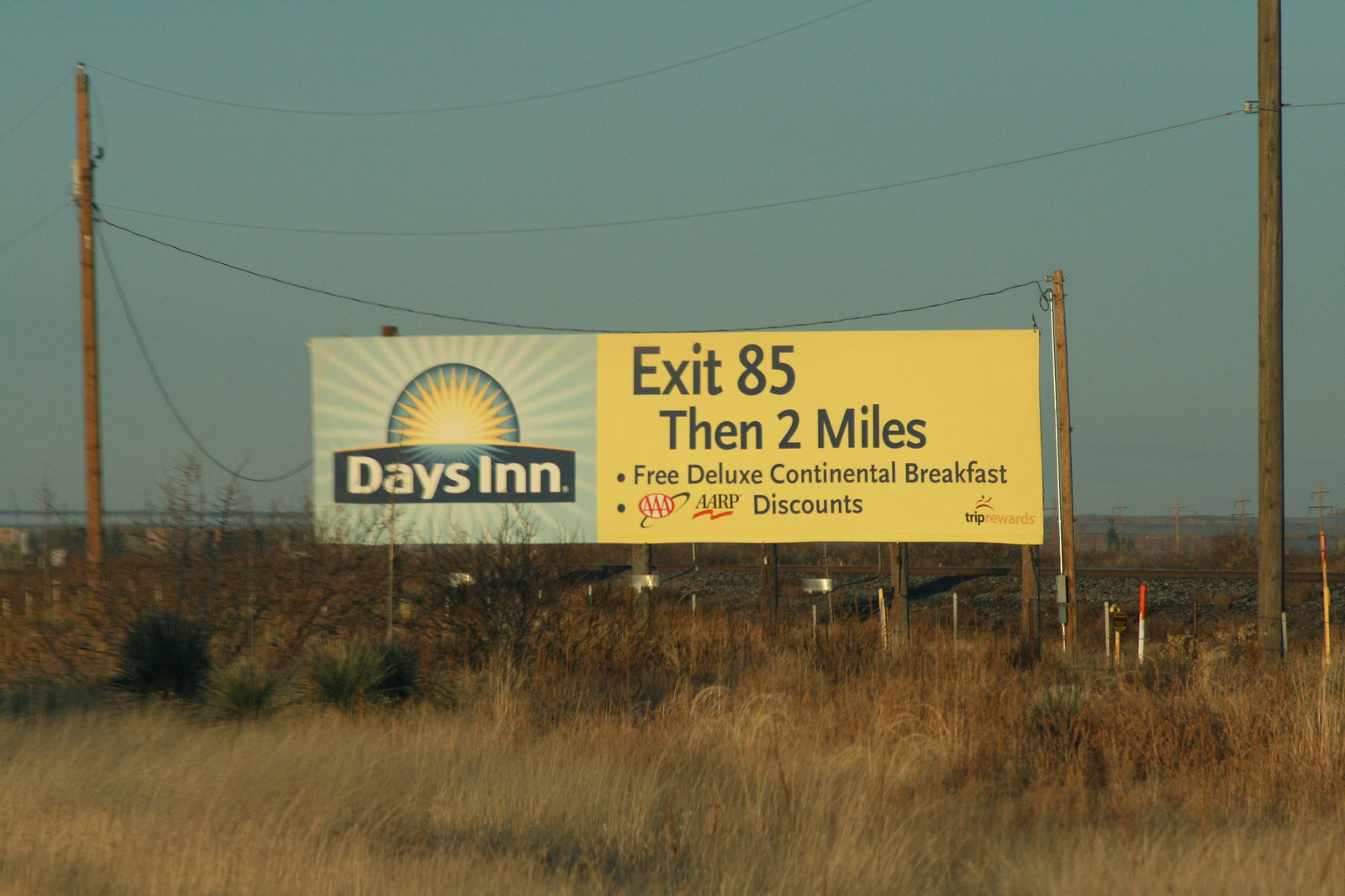This image captures a bright outdoor scene depicted in a square format. The sky forms a serene backdrop with its light blue color, stretching across the top part of the image. Prominently positioned in the middle is a large, rectangular billboard, divided into two distinct sections.

The left side of the billboard features a light blue background with a cheerful illustration of a shining sun, rendered in yellow and white hues. Below the sun image, the text "DAYS INN" is spelled out in clean, white letters.

On the right side, the billboard's background shifts to a vibrant yellow. Bold, black text commands attention, starting with "EXIT 85" at the top, followed by "2 MILES," and concluding with "FREE DELUXE CONTINENTAL BREAKFAST," enticing travelers with its inviting offers.

The detailed combination of colors and information effectively attracts the viewer’s eye, making the billboard a standout feature in this outdoor setting.